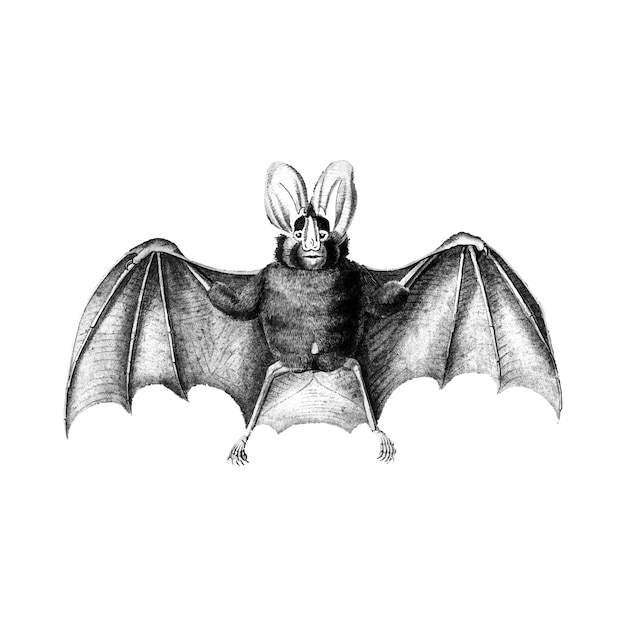The image is a black and white sketch of a bat with its wings sprawled wide open, revealing intricate details of its arms, legs, and the delicate bones within its wings. The bat is positioned facing forward, much like the iconic Batman logo, giving a clear view of its distinct features. Its head features a long-shaped mouth, a triangular nose, chubby cheeks, small eyes, and exceptionally large, grape-shaped ears that are lighter in color, likely white or light grey. The bat sports a plump stomach area and its body is predominantly black fur with some white and grey tones. The sketch portrays the bat as having a funny, smirking expression, creating a unique, almost whimsical character. The plain white background emphasizes the detailed and symmetrical depiction of the bat.